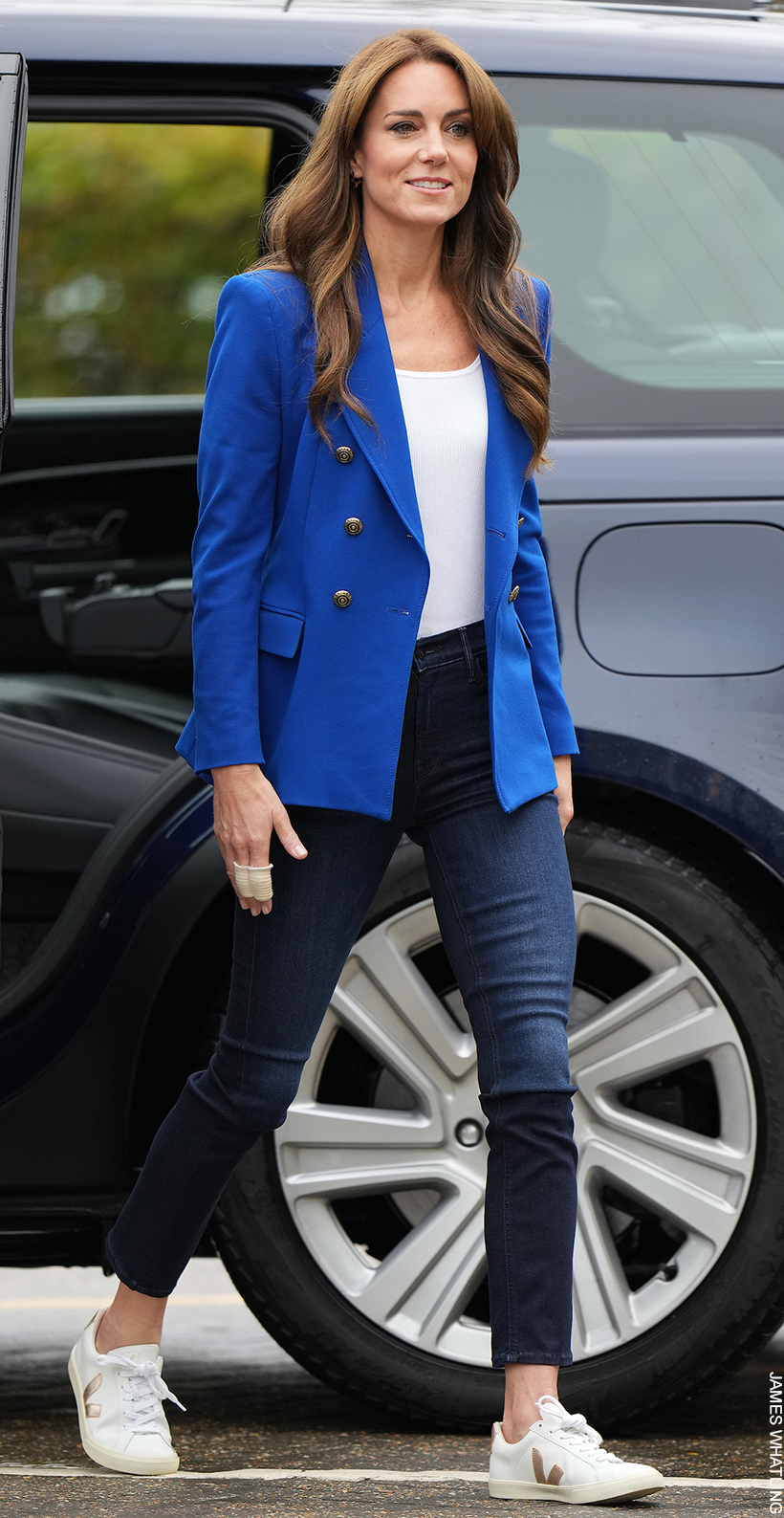The image captures Kate Middleton, stepping out of the back driver’s side of a large gray SUV with white hubcaps. The SUV's interior is also a matching shade of gray. Kate is smiling warmly, showing her teeth, suggesting she is in a happy mood. Her long, curled and waved hair, a brownish blonde in color, cascades down as she moves. She is wearing a stylish ensemble featuring a white undershirt layered beneath a blue blazer adorned with three silver buttons, and dark, tapered denim jeans. Her footwear consists of white and gold tennis shoes. Notably, she has a bandage wrapped around her right hand’s index and middle fingers. The image is closely focused on her, emphasizing the details of her attire and expression, while a greenish blur through the SUV windows hints at natural scenery in the background. Only a small portion of the road is visible at the very bottom of the picture, as Kate spans the entire height of the frame, captured mid-step with the back tire positioned behind her.